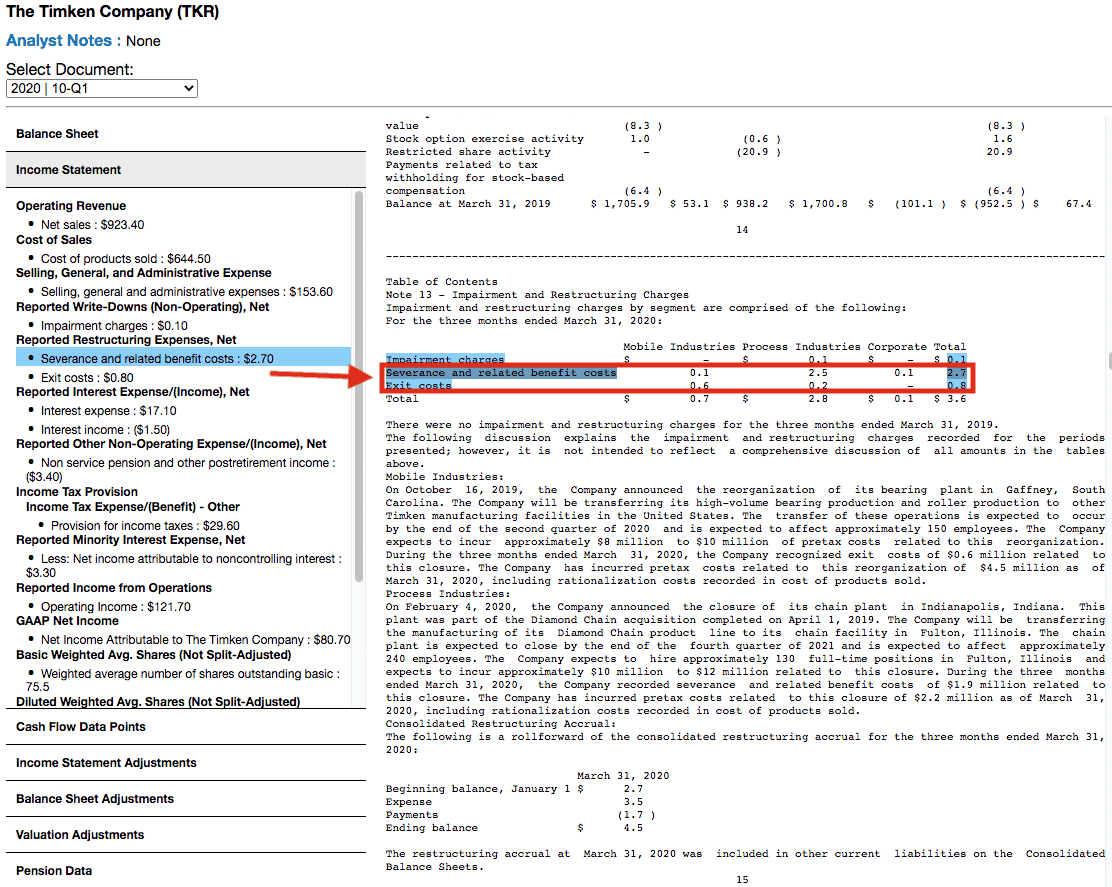**Detailed Caption:**

The screenshot displays a data table from The Timken Company, denoted as 'TKR'. At the top left of the screenshot, “The Timken Company (TKR)” is prominently labeled. Beneath this, the term "Analyst Notes" is shown with an indication that no notes are available. Further down, there's a dropdown menu labeled "Select Document," currently set to "2020-10-Q1."

The main section of the table starts with "Balance Sheet" and "Income Statement" headers, followed by detailed financial entries under various categories. The "Operating Revenue" section lists the net sales figure as 923.40. The "Cost of Sales" is broken down with "Cost of Products Sold" listed at 644.50. The "Selling, General, and Administrative Expense" is 153.60. Following this, "Reported Write Downs, Non-Operating Net Impairment Changes or Charges" is noted at 0.10. The "Reported Restructuring Expenses" category shows "Severance and Related Benefit Cost" at 2.70.

A notable feature on the page is a red arrow pointing to the right side of the screen, where a red rectangle encloses two items: "Severance and Related Benefit Cost" and "Exit Cost." Within these categories, various figures are listed under different labels. Specifically, "Industries" is broken down into sub-entries with values 0.1 and 0.6. Another "Industries" entry lists 2.5 and 0.2. In the "Corporate" section, only Severance is noted with a figure of 0.1. The cumulative total under "Severance and Related Benefit Cost" is 2.7, while the total for "Exit Cost" is 0.8.